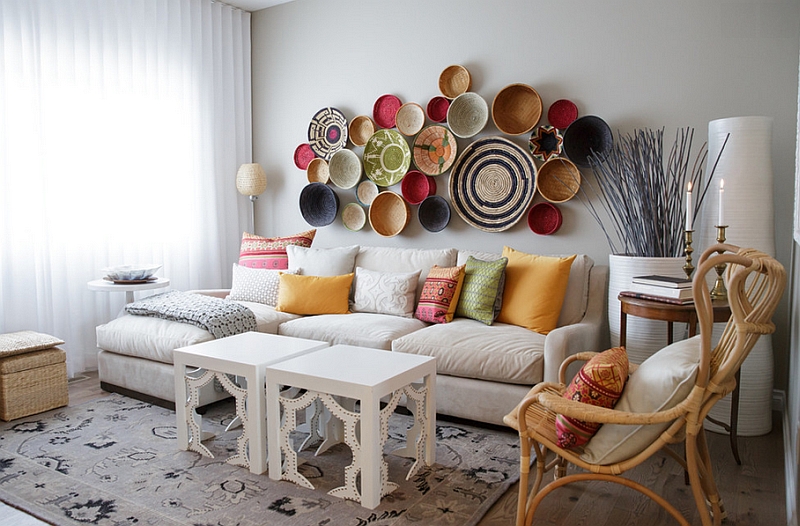The image presents a well-lit and brightly colored living room scene. Central to the image is a white sofa adorned with vibrant pillows in shades of golden, green, pink, red, orange, and white. In front of the sofa, there is a leg stool draped with a black and grey blanket, accompanied by two small white rectangular tables. To the right of the scene stands a brown wooden chair featuring two additional pillows. The left side of the image is defined by a white curtain, beside which a lamp is placed in the corner. The wall above showcases a stunning array of decorative bowls, exhibiting a variety of colors including brown, blue, white, green, orange, and black, all with unique patterns. Near the sofa, there is a table holding some books and candles. A rug covers the floor, further enhancing the cozy ambiance of the room. The photo is clear, with excellent image quality, ensuring that all details are easily visible.